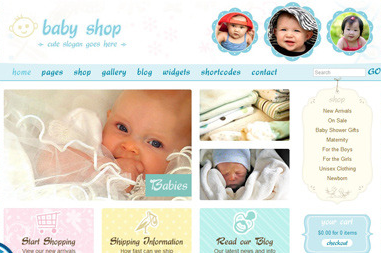This is a small image of a baby shop website template featuring a minimalist white background. At the top left corner is the company logo, a charming yellow baby face illustration accompanied by the text "Baby Shop" in light blue. Directly beneath this, a placeholder slogan reads, "Cute Cute Slogan Goes Here." 

To the right of the logo are three small images of babies, each encased in a flower-shaped border. Below these images lies the navigation menu, which sports a light blue background and dark blue text. The menu options read: Home, Pages, Shop, Gallery, Blog, Widgets, Short Codes, Contact, and include a search bar.

The main content area displays a large image of a baby, flanked by two smaller images. Adjacent to these images is a promotional section highlighting key categories: "Shop New Arrival," "On Sale," "Baby Shower Gifts," "Maternity," "For the Boys," "For the Girls," "Unisex Clothing," and "Newborn."

Below this section are three call-to-action windows: the first window, with a pink background, reads "Start Shopping;" the second, with a yellow background, is labeled "Shipping Information;" and the third, with a bluish background, invites visitors to "Read Our Blog." At the bottom right corner, a small blue button provides quick access to the shopping cart and checkout process.